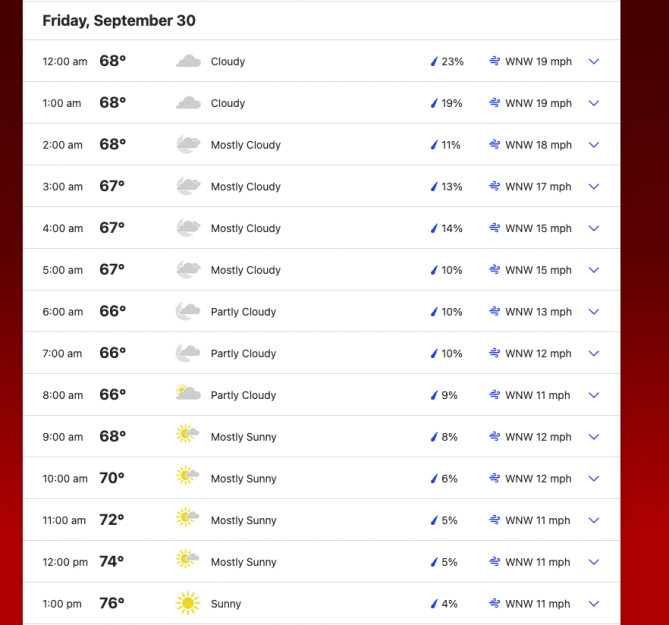The image presents a detailed weather forecast displayed on a red gradient background. The gradient transitions from a dark, deep red at the top to a brighter royal red towards the bottom. Within this background, there's a rectangular section with a white backdrop, framed by a light, thin gray border at the top.

At the top-left corner, bold black lettering announces "Friday, September 30". Directly beneath this, a gray line serves as a divider. Below the line, in small gray letters, the time "12:00 AM" is indicated. Following the time, in bold black numbers, the temperature is displayed as "68°". Adjacent to this, a gray cloud icon signifies "Cloudy" weather conditions. To the right of the cloud, a raindrop symbol indicates a 23% chance of precipitation. Further right, a blue wind symbol shows "WNW" (West-Northwest) wind direction at 19 mph. An interactive blue arrowhead pointing downwards indicates more information is accessible via a dropdown menu.

Following another gray divider, the schedule continues with "1:00 AM" written in small black letters. To the right, the temperature "68°" is presented in a bold, rounded sans-serif font. The weather condition is marked as "Cloudy" again, with a corresponding gray cloud icon. To the right, a raindrop symbol shows a decreased 19% chance of precipitation. Adjacent to this, another blue wind symbol denotes "WNW" winds at 19 mph. The blue dropdown menu arrowhead is also present here for further details.

A subsequent divider separates this segment from the next update at "2:00 AM" in small lettering. The temperature remains at "68°", shown in the same bold, rounded font. This forecast features a gray crescent moon partly obscured by a light gray cloud, indicating "Mostly Cloudy" conditions. The probability of precipitation has dropped to 11%, as depicted by a raindrop symbol. The blue wind symbol once again specifies "WNW" wind direction, but now at 18 mph. The interactive blue arrowhead persists, pointing downwards for additional information.